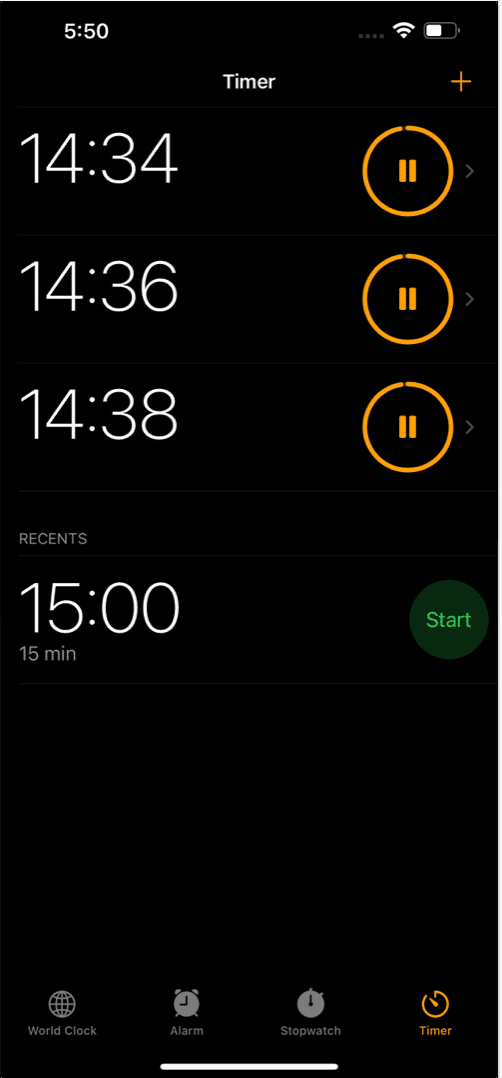The image is a screenshot of a cell phone displaying the timer feature. In the upper right-hand corner, the battery indicator, signal strength indicator, and timestamp confirm this is a mobile device. The center of the screen prominently displays the word "Timer" in white font. Below this title are three elapsed times: 14 minutes and 34 seconds, 14 minutes and 36 seconds, and 14 minutes and 38 seconds, likely representing intervals being tracked.

Further down, there's a section labeled "Recents," featuring an upcoming 15-minute timer. This timer is ready to be initiated, signified by a large green start button next to it. The bottom part of the screen includes four icons, each corresponding to different functions within the timer system. The overall setup indicates that the user is meticulously timing various activities.